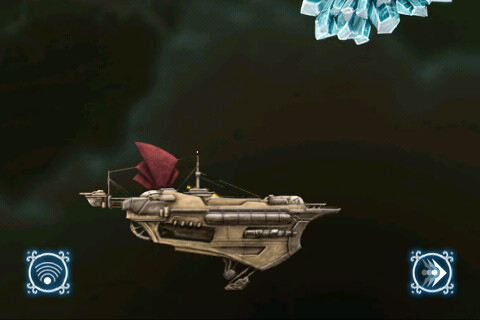The image appears to be a scene from a steampunk-themed game, showcasing a detailed side view of a ship floating in a non-aquatic environment. The ship, resembling a vintage steam-powered vessel, is predominantly beige and bronze with intricate metallic components adorning its edges. Various wires emerge from the ship, connecting to a pole-like structure that is also adorned with red flags. The background is a blend of beige, gray, black, and hints of green, creating a somewhat muted, otherworldly atmosphere. In the top right corner, there is a crystal-like shape emitting a blue hue, adding a mystical element to the scene. The bottom left corner features a circular symbol reminiscent of a Wi-Fi icon, while the bottom right corner hosts another circle containing arrow-like designs.